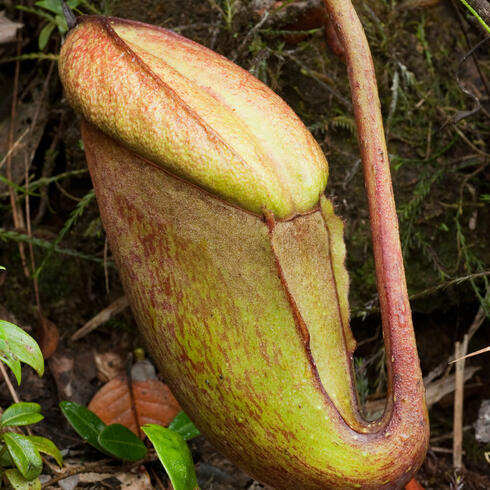The photo depicts a large, exotic plant positioned outdoors among a carpet of green leaves, sticks, and soil. The central feature of the plant is a striking, pitcher-like structure, blending light green-yellow hues with patches of red. It has a unique teapot-like shape with a distinctly long tube or tail-like extension on the right side, curving upwards. Although the day is overcast, which lends a muted light to the scene, the plant's vibrant colors stand out against the forest floor comprised of both green foliage and brown, fallen leaves. The plant's base is green with a red stem, suggesting it could be a tropical pitcher plant, perhaps designed to capture insects. Its intriguing form and colorful appearance give it an almost otherworldly presence amid the natural forest setting.